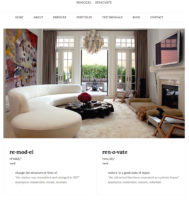The image depicted is of a modern living room with several stylish design elements, though it suffers from poor resolution that makes the text within it illegible. The background is white, with two indistinct words positioned centrally on the upper portion, followed by a navigation strip containing seven words. Below this, a photograph showcases a contemporary living room setup. The room features a distinctive, curvaceous white couch that forms a circular end, paired with a low, black, tire-like coffee table. Mounted on the white wall above the white fireplace is a flat-screen TV, and a white circular chandelier hangs from the ceiling. Behind the sofa is a large, multicolored piece of art, and the background reveals windows and doors leading out to a balcony. Additionally, there are two sections below the living room image, each containing a dark black header with text below, similar in size and shape, though unreadable due to the blurriness.